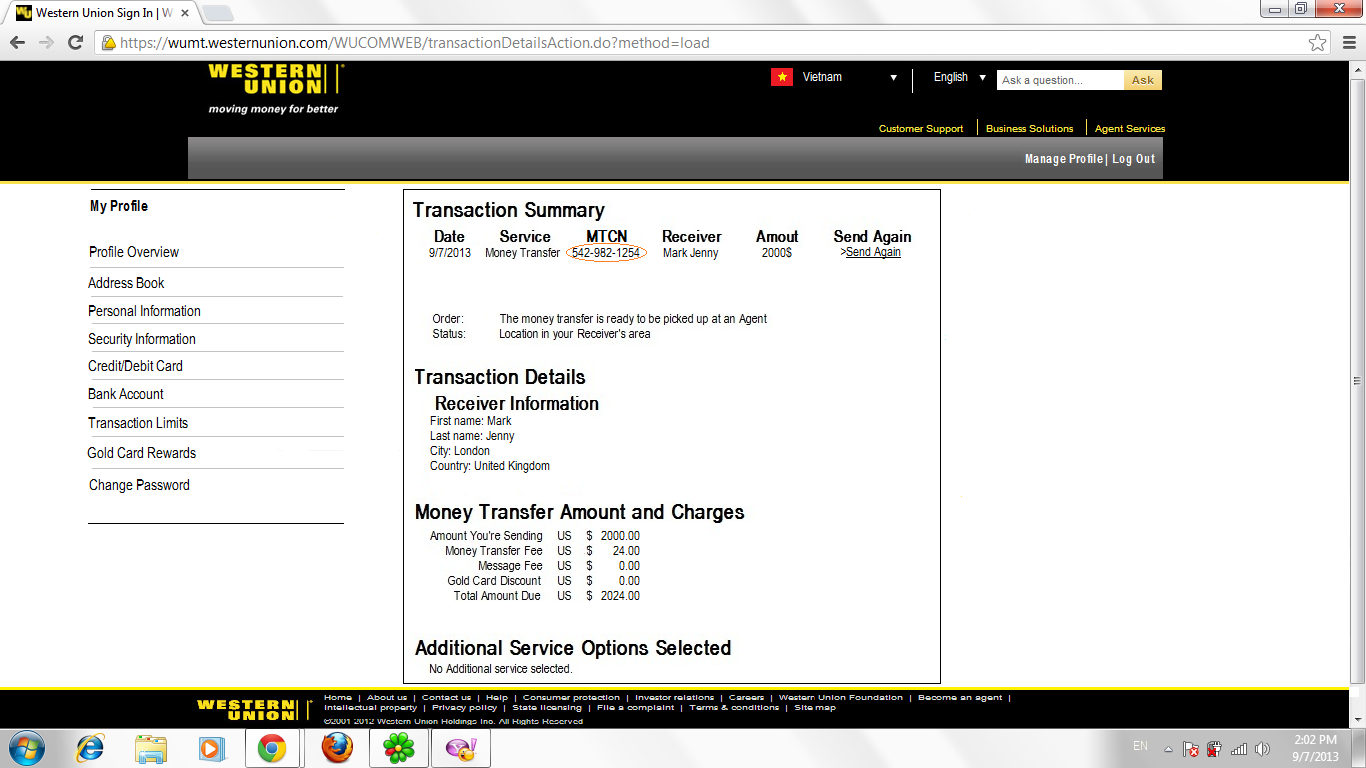This screenshot, presented in landscape mode, captures the Western Union sign-in page. In the upper left-hand corner, the page's tab indicates it belongs to the Western Union website. Adjacent to this, the upper right-hand corner displays a red 'X' close button. Below these elements, the URL bar confirms the site as "wmt.westernunion.com". 

The next row features a prominent black stripe adorned with the Western Union logo and the slogan "Moving Money for Better." Adjacent to this, the Vietnamese flag is visible, implying that the user might be Vietnamese or prefers Vietnamese despite English being selected. To the right of the flag, there is a search bar prompting the user to "Ask a question."

Underneath the stripe, navigation links including "Customer Support," "Business Solutions," and "Agent Services" are available. Below these links, a large gray stripe spans the screen, featuring options to "Manage Profile" or "Log Out" on the right-hand side.

The main portion of the screenshot divides into two columns. The left column lists several user options: "My Profile," "Profile Overview," "Address Book," "Personal Information," "Security Information," "Credit/Debit Card," "Bank Account," "Transaction Limits," "Gold Card Rewards," and "Change Password."

The right column displays transaction details, where a small circle highlights the section under "Transaction Summary." Here, the date "9-7-2013" is listed alongside "Service: Money Transferred." The circled number, "MTCN: 542-982-1254," identifies the specific transaction. The receiver, "Mark Jenny," is set to receive $2,000, with an option to send the amount again. The order summary indicates that the money is ready for pick-up at an agent in the receiver's location, London, UK. Additional transaction details include the transfer fee of $24. This screenshot likely serves to assure the receiver, Mark Jenny, that the money is prepared for collection.